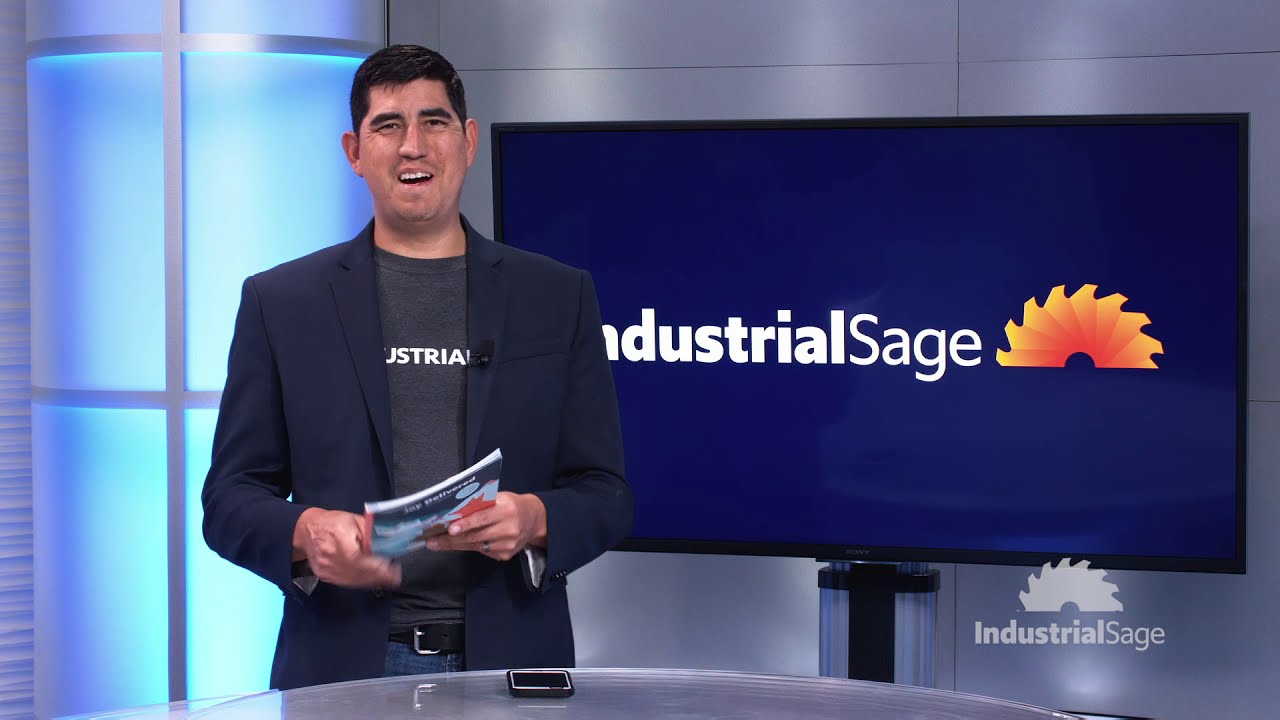The image depicts a TV anchor in an indoor setting, standing on the left side. This light-skinned gentleman has very dark black hair, black eyebrows, and an oval-shaped face with ears that poke out slightly. His mouth is open, revealing the top of his teeth, and he wears a dark gray sports jacket over a gray t-shirt adorned with partially visible white lettering, "USTRIA." A microphone is clipped to his jacket lapel. He holds what appears to be a book or magazine in his hands. In front of him is a circular glass table with a cell phone placed on top, obscuring the lower part of his body. To his right, a large TV screen on a gray wall displays the words "Industrial Sage," with some letters partially obscured by his shoulder. The screen features an orange and yellow table saw design, with a similar icon in white underneath the text. Behind him on the left side of the screen, a cylindrical structure with blue lights and gray grids is also visible. A watermark in the bottom right corner of the screen reads "Industrial Sage."